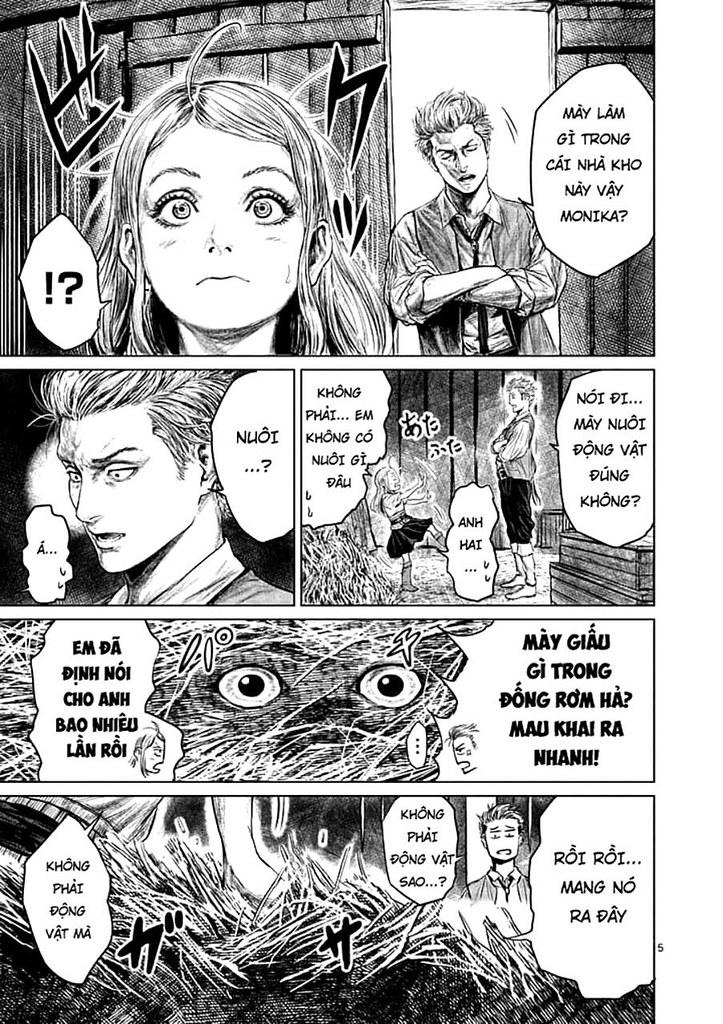This black and white comic book page features a series of frames, each varying in size. The largest frame is at the top, depicting a surprised woman in the foreground, represented by a thought bubble with a question mark and exclamation point. Behind her to the right, a stern-looking man stands in a doorway. The dialogue in their speech and thought bubbles is in Thai, with some bolded lettering for emphasis. The subsequent frames show interactions between the man and woman, indicating a tense conversation. The man is often depicted with furrowed brows, appearing angry or stern, while the woman looks frightened. One panel zooms in on just a pair of eyes, intensifying the scene's emotion. The bottom frame introduces a monster-like character amid what looks like hay or grass, with a dubious expression from the man while the woman is no longer visible.